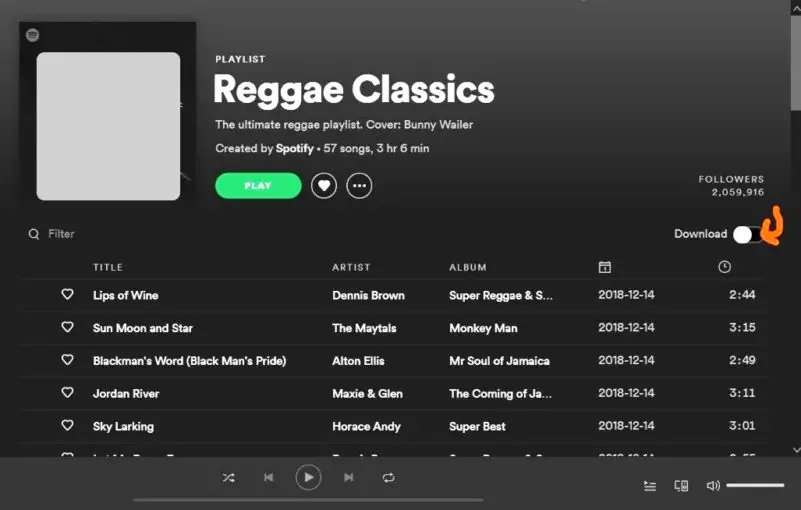Here is a cleaned-up and detailed caption:

---

Screenshot of a Spotify playlist titled "Reggae Classics." The playlist is hailed as the Ultimate Reggae Playlist and features an image of Bunny Wailer on the cover. Curated by Spotify, it comprises 57 classic reggae tracks spanning a total duration of 3 hours and 6 minutes. Dominating the view is a large play button, inviting listeners to dive into the collection.

Highlighted tracks from the list include:
1. "Lips of Wine" by Dennis Brown
2. "Sun, Moon, and Stars" by The Maytals
3. "Monkey Man" by The Maytals
4. "Black Man's Pride" by Alton Ellis, featured in the album "Mr. Soul of Jamaica"
5. "Jordan River" by Maxine Glynn
6. "The Coming of Jah" by Horace Andy

All songs were added on December 14, 2018. The Spotify interface is set against a sleek black background, adding to the playlist's timeless appeal.

---

This detailed description offers a comprehensive view of the playlist, enhancing the reader's understanding of its content and presentation.